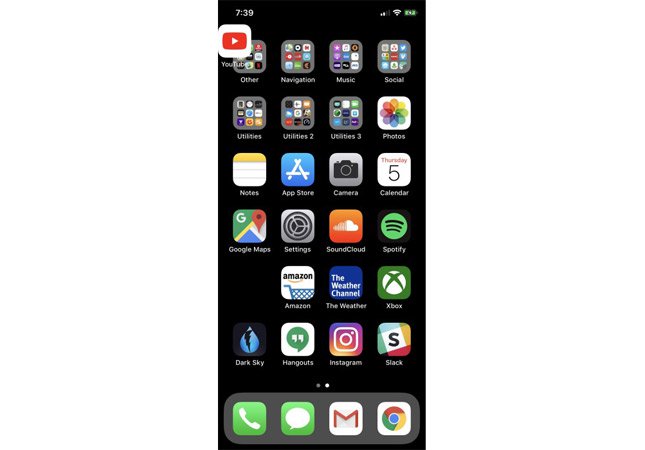This image appears to be a screenshot of a smartphone's home screen, set against a black background. The most prominent feature is the YouTube app icon, which looks as if it is in the process of being moved. In the top-left corner of the screen, the status bar shows the current time as 7:39 and the battery icon indicates a full charge.

The home screen displays several categorized folders. At the top, there are folders labeled Navigation, Music, Social, and three separate Utility folders. In addition to these folders, individual app icons are organized neatly in rows. These include Photos, Notes, App Store, Camera, Calendar, Google Maps, Settings, SoundCloud, and Spotify. There is an empty space where the YouTube icon might soon be placed. Following this, the app icons for Amazon, Weather, Xbox, Dark Sky, Hangouts, Instagram, and Slack are displayed.

At the bottom of the screen, the dock contains four frequently used apps: the Phone app depicted with a green call button, the Messaging app also indicated by a green message bubble, the Gmail app, and the Chrome browser icon.